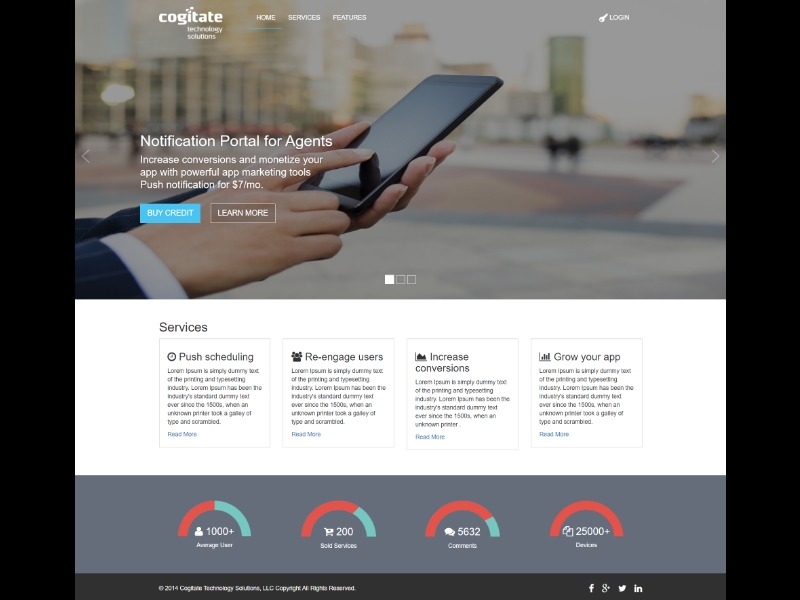The image is a colorful screenshot of the Cogitate Technology Solutions website, viewed on a computer. The brand name "Cogitate" is displayed in lowercase text. The website features a navigation bar with three tabs: "Home," "Services," and "Features." The user is currently on the Home tab. On the right-hand side, there is an option to log in, indicating that the user is not yet logged into the portal. 

Prominently displayed in the center of the page is a title that reads, "Notification Portal for Agents." Below this, a tagline encourages users to "Increase conversations and monetize your app with powerful app marketing tools." The portal offers push notifications starting at $7 a month, with options to purchase credits or learn more.

Further down, the site details various services such as push scheduling, user re-engagement, conversation increases, and app growth. At the bottom, the website displays impressive statistics, including "1,000+ average users" and "200 sold services," among others.